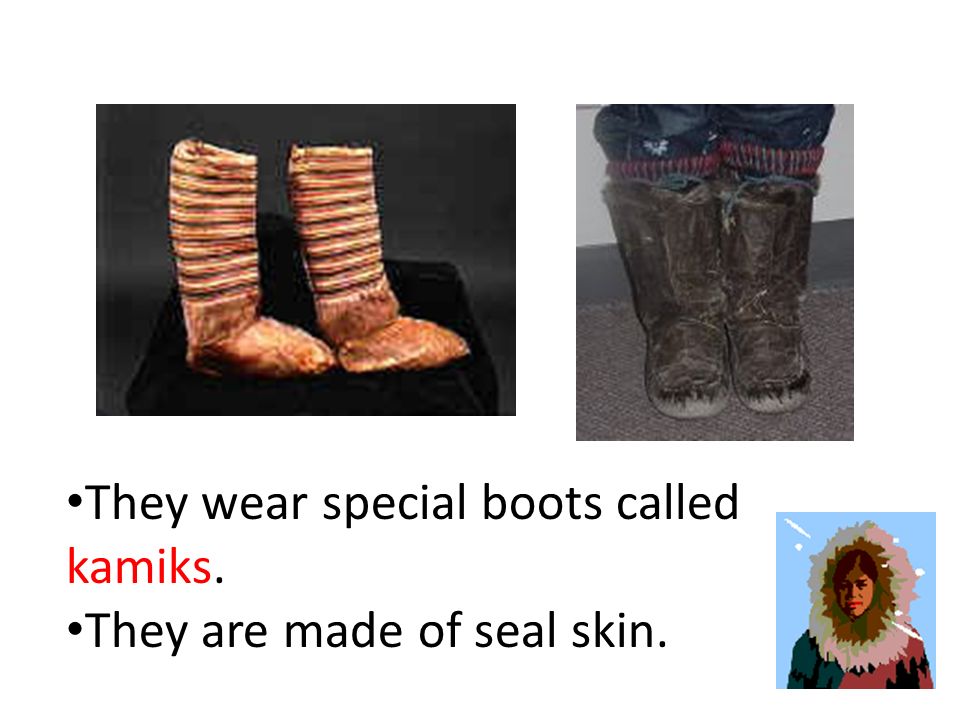This image, arranged in a landscape orientation, presents a carefully arranged infographic showcasing traditional Eskimo footwear and attire alongside descriptive text. At the upper left, a pair of ancient, museum-displayed knee-length boots in dark beige with lighter beige horizontal bands sit on a black pedestal. Adjacent to these, on the right, are modern yet traditionally styled dark brown boots, adorned with elaborate black designs and a red band around the top, worn over jeans with a sandy ground beneath. Below the boots, a textual description in two bulleted points reads, "They wear special boots called kameks," with the term 'kameks' highlighted in red, and continues, "they are made of sealskin." Complementing these visuals, in the bottom right corner, there's a digitized illustration of an Eskimo woman, her face framed by a fur-lined hood, set against a light blue background, signifying the sky. The woman's maroon coat with black accents adds further cultural context. The graphic merges these color photographs and digital illustration with clear typography, evoking a structured, PowerPoint presentation style.